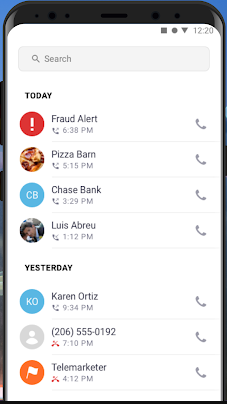The image features a screenshot of a call log from a smartphone. At the very top of the screen, there is a search bar. Below the search bar, the call log is divided into sections labeled "Today" and "Yesterday."

In the "Today" section, the calls are listed in the following order:

1. Fraud Alert
2. Pizza Barn
3. Chase Bank
4. Louise Abera

The timestamps for these calls range from 6:38 PM to 1:12 PM.

In the "Yesterday" section, the calls are listed as follows:

1. Karen Ortiz
2. A phone number: 206-555-0192
3. Telemarketer

The timestamps for these calls range from 9:34 PM to 4:12 PM.

The detailed call times and contacts highlight the frequency and variety of incoming and outgoing calls on the device.